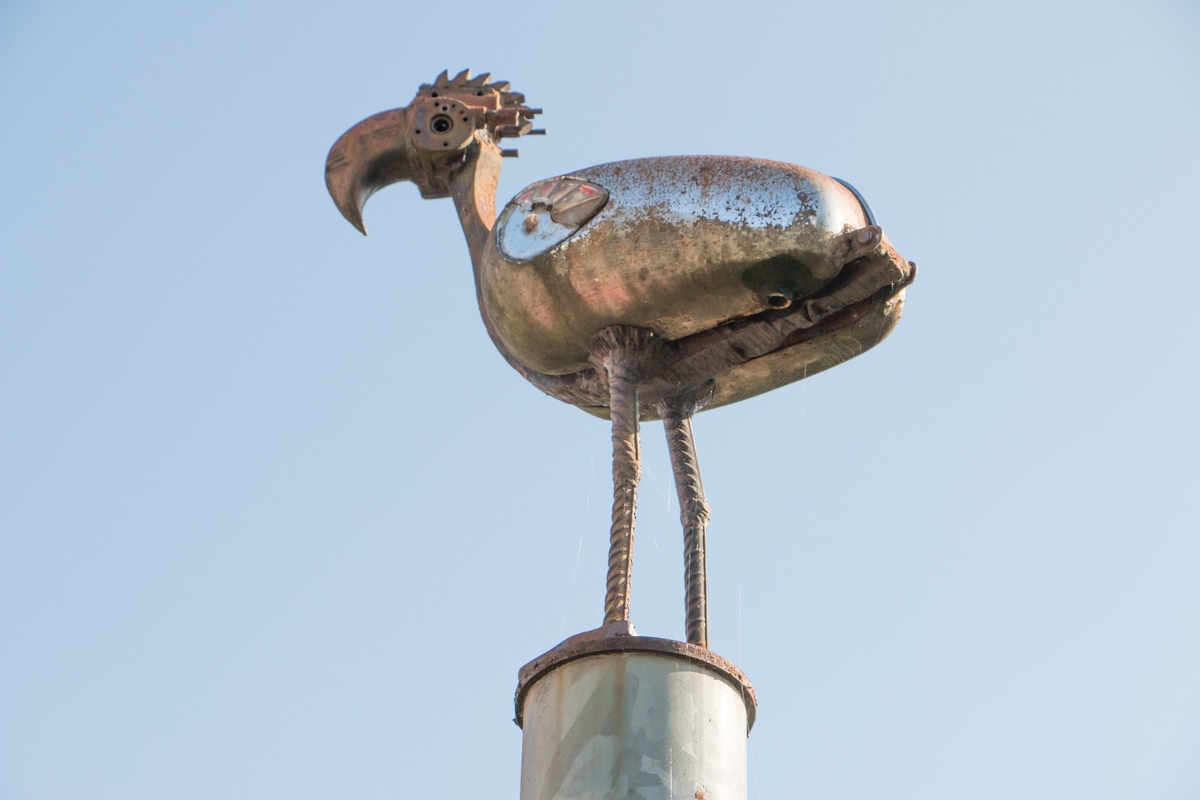The image depicts a bronze-colored metal statue of a bird, which looks like a weather vane, set against a light blue sky background. The bird features a long, slightly downward-angled beak reminiscent of a crochet hook, small stick-up feathers on its head, and a distinctive black eye surrounded by a few holes. Its body exhibits a blend of bronze and light blue, possibly spray-painted, giving it a slightly rusty and aged appearance. The bird is perched on a round, metal cap that sits atop a vertical cylinder or smokestack, which is similarly rusty and dirty white in color. The bird’s long, thin legs, adorned with a rope-like pattern, give it an airy, delicate stance isolated against the serene sky.